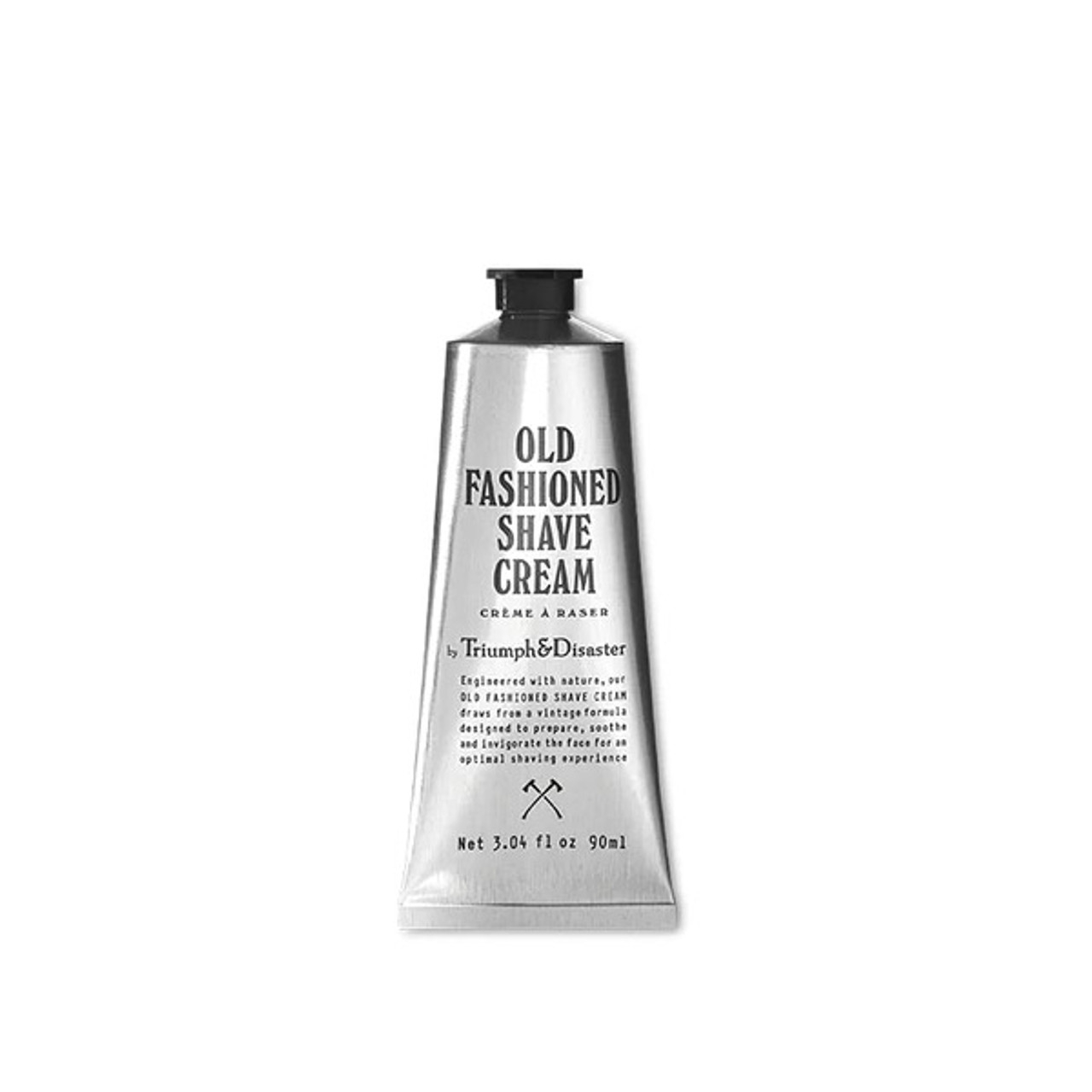The image features a digitally edited product photo of a vintage-inspired, unused silver tube of "Old-Fashioned Shave Cream" by Triumph and Disaster, set against a clean white background. The reflective tube, resembling a shorter, more tapered version of a toothpaste tube, is adorned with detailed text highlighting its key features: "Triumph and Disaster," "engineered with nature," and specifics on its soothing, invigorating shaving formula. The black screw-type lid contrasts sharply with the silver body of the tube, which proudly displays the net weight of 3.04 fluid ounces (90 milliliters). Notably, the design includes a distinctive logo of two crossed axes near the bottom, emphasizing its rugged, yet refined appeal.